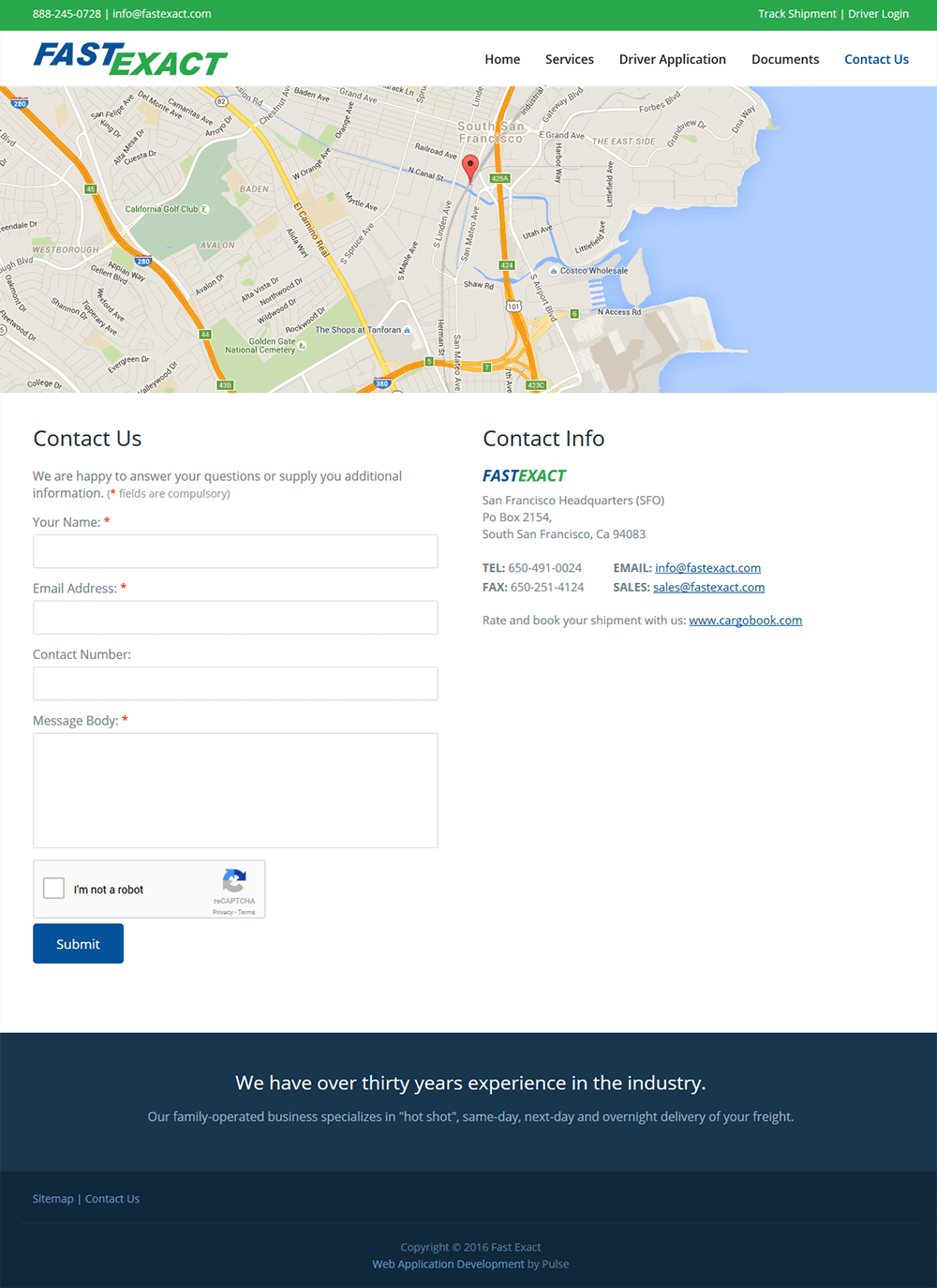This is a detailed description of the Contact Us page:

The Contact Us page is captured in a screenshot showcasing a sleek and user-friendly interface. At the top, a green bar draws attention with the message and contact information including a phone number and an email address. The logo of the company prominently features "Fast" in blue and "Exact" in green.

To the right of the logo, a navigation bar is present, including the options: Home, Services, Driver Application, Documents, and Contact Us. The "Contact Us" link stands out in blue, while the other four links are displayed in black.

A large map with an icon enhances the page, pinpointing the location relevant to the contact information. Below the map, a standard contact form is available for users to fill out. The fields include Name, Email, Contact, and Message Body, followed by a "I'm not a robot" CAPTCHA for security. A blue "Submit" button completes the form for user interaction.

To the right side of the form, the Contact Info section provides the details, including the company's logo, the address of the San Francisco Headquarters, a telephone number, and an email for sales inquiries.

The footer at the bottom of the page is a distinguished navy blue, containing a brief statement: "We have over 30 years experience in the industry," emphasizing the company’s long-standing expertise and reliability.